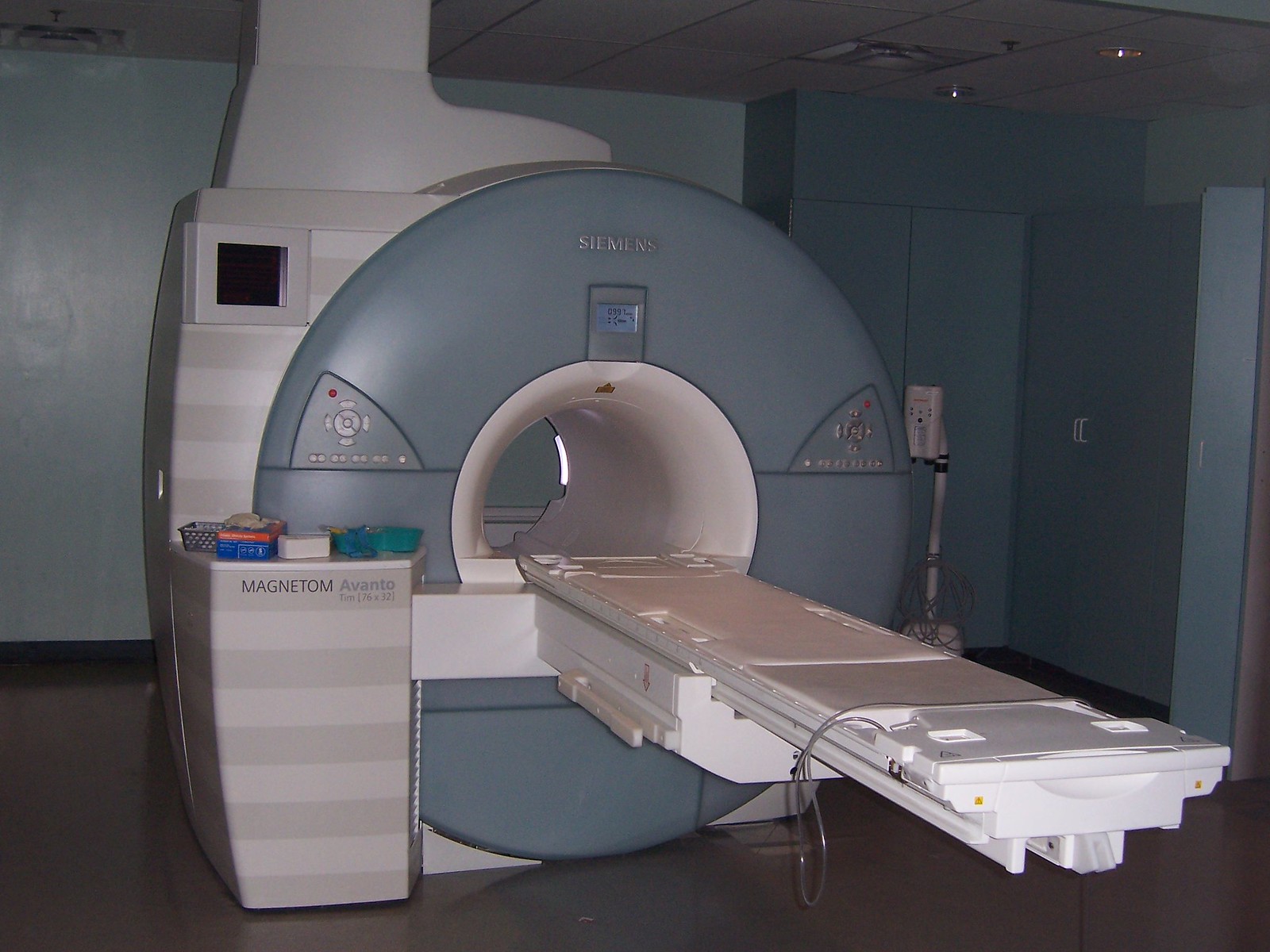The photograph captures a detailed side view of a Siemens medical imaging machine, likely used for MRIs or CAT scans. The central component of the machine features a large, rounded, donut-like structure with a silvery blue exterior and a white center. Prominently, the Siemens logo is located at the top of this rounded section. A beige shelf extends from the side of the donut-shaped core, labeled "Magnetom Avanto 76 by 32." The machine includes a flat, white table or stretcher intended for the patient, which slides into the central arch of the imaging apparatus. On either side of the machine, there are operational buttons and a control screen positioned at the top.

The room surrounding the machine includes blue cupboards on the right side, with the back wall and other elements of the room also predominantly blue. The ceiling is white, equipped with dim yellow lights and gray vents, contributing to the clinical ambiance. The floor in the room is dark, contrasting with the lighter elements of the room, creating a typical hospital setting. The detailed machinery and organized layout signify a functional and well-equipped medical imaging environment.